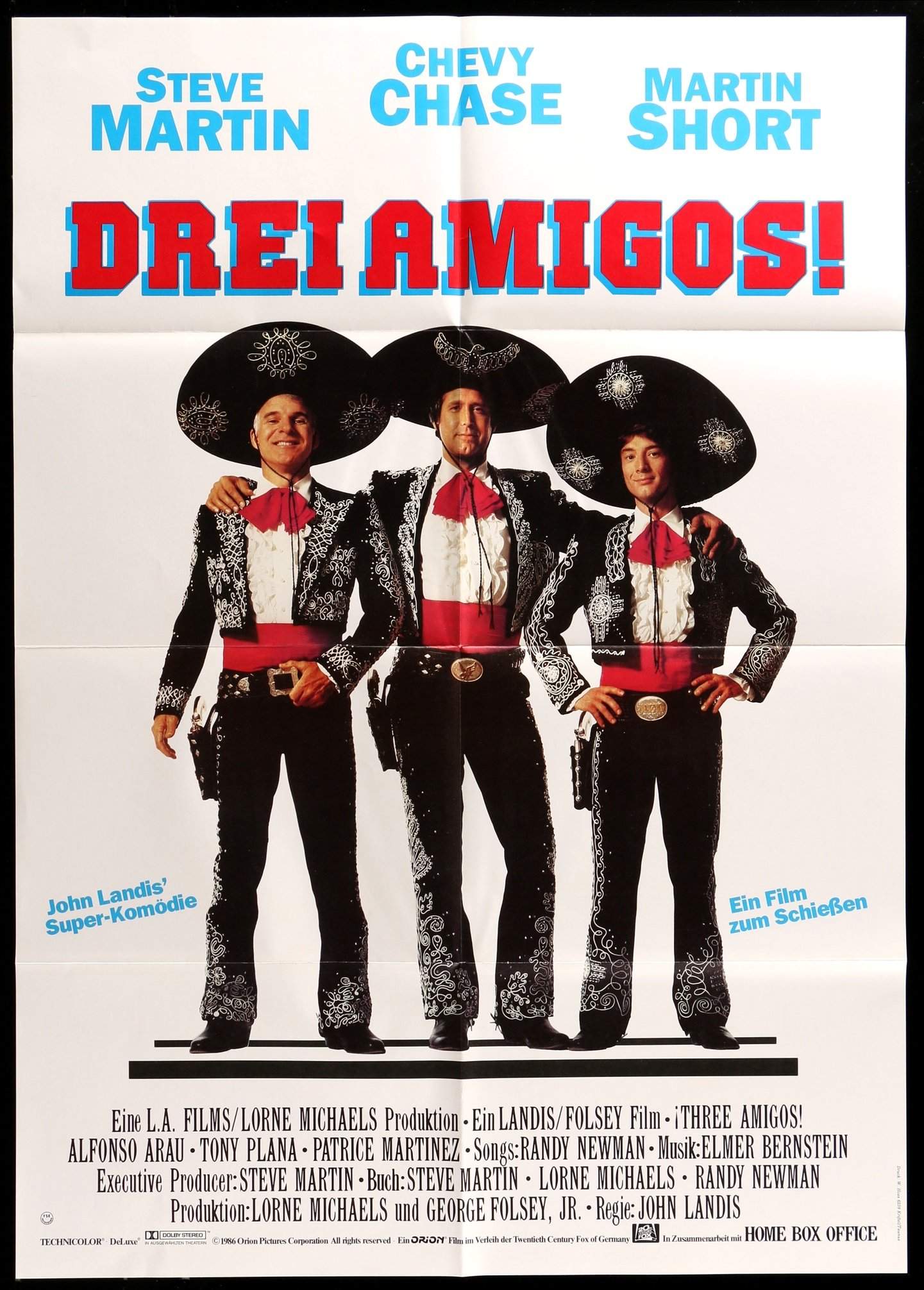This image is a German-language movie poster for the classic 1980s comedy "The Three Amigos." Dominated by a white background, the top features the names "Steve Martin, Chevy Chase, Martin Short" in light blue text. Just below this, in bold red uppercase text with a blue backdrop, it reads "DREI AMIGOS." Central to the poster are the three actors—Steve Martin to the left, Chevy Chase in the middle with his arms around his co-stars, and Martin Short on the right. They are all smiling, dressed in traditional mariachi outfits. The outfits include large black sombreros adorned with white floral trim, black mariachi suits with red and white detailing, gold belt buckles, and red sashes tied around their waists. In the center portion of the poster, on the left, it reads "John Landis, super Komödie," and on the right, "Ein Film zum Scheiben," indicating the director and film type. At the bottom, there is a list of credits mentioning "LA Films, Lorne Michaels production, Landis/Bosby Films," highlighting the producers and production companies involved.